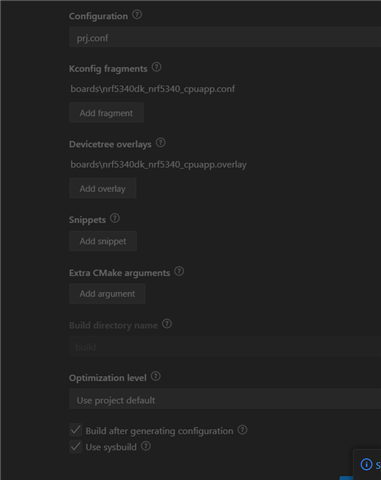The image displays a command interface on a computerized system with a predominantly black background and text in a light grayish-white color. The interface is divided into several sections with each section providing functionalities and options for configuration.

1. **Configuration**: This section has a title "Configuration?" centered within a circle. Below it is a bar labeled "PRJ.CONF."

2. **Kconfig Fragments**: The title "Kconfig Fragments?" is displayed with a question mark centered within a circle. Beneath it, there is a path "board/nrf5340dk_nrf5340_CPUAPP.CONF" and a square button labeled "Add Fragment."

3. **Device Tree Overlays**: The title "Device Tree Overlays?" is shown with a question mark centered within a circle, similar to the previous sections. The path "board/nrf5340dk_nrf5340_CPUAPP.overlay" is displayed with a square button labeled "Add Overlay."

4. **Snippets**: This section is titled "Snippets?" with a circle containing a question mark in the center. There is a gray button labeled "Add Snippet."

5. **Extra CMake Arguments**: "Extra CMake Arguments?" is the title here, with another circular question mark. There is an option to add an argument within a gray box.

6. **Build Directory Name**: This section features the title "Build Directory Name" with a box containing the word "build," which is visible but not highlighted.

7. **Optimization Level**: Here, the title "Optimization Level?" is displayed with a centered question mark within a circle. The text says "Use Project Default."

At the bottom of the interface, there are two options with corresponding white checkboxes:
- "Build after generating configuration"
- "Use sys build"

Each of these sections and options allows for specific modifications and settings to be configured within the software environment, providing a comprehensive and detailed system configuration tool.